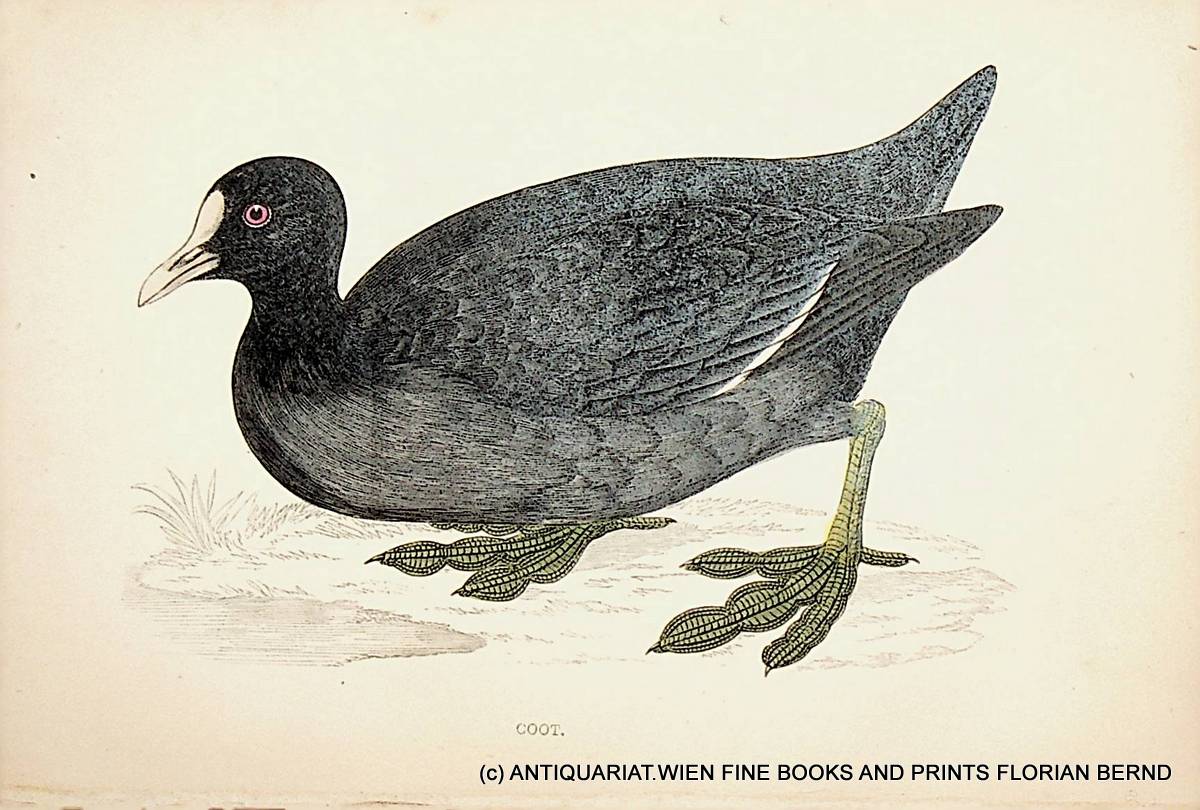In the image, there is a detailed drawing of a black duck with strikingly large, yellow webbed feet that appear oversized compared to its body. The bird is in a crouched position, leaning to the left, with its head also turned left. Its plumage is primarily black and gray, with a speckled, salt-and-pepper effect on the tips of its tail feathers. The beak is a whitish cream color, and the duck has a distinctive eye with a black pupil encircled by a red ring. The background suggests a natural setting with hints of water and grass, including a notable patch of taller grass. The artwork is rendered on light tannish, slightly yellow-tinted paper. At the bottom right corner, the text reads "COOT." followed by "(c) Antique WE Fine Books and Prints Florian Byrne," indicating the copyright and the artist's details.